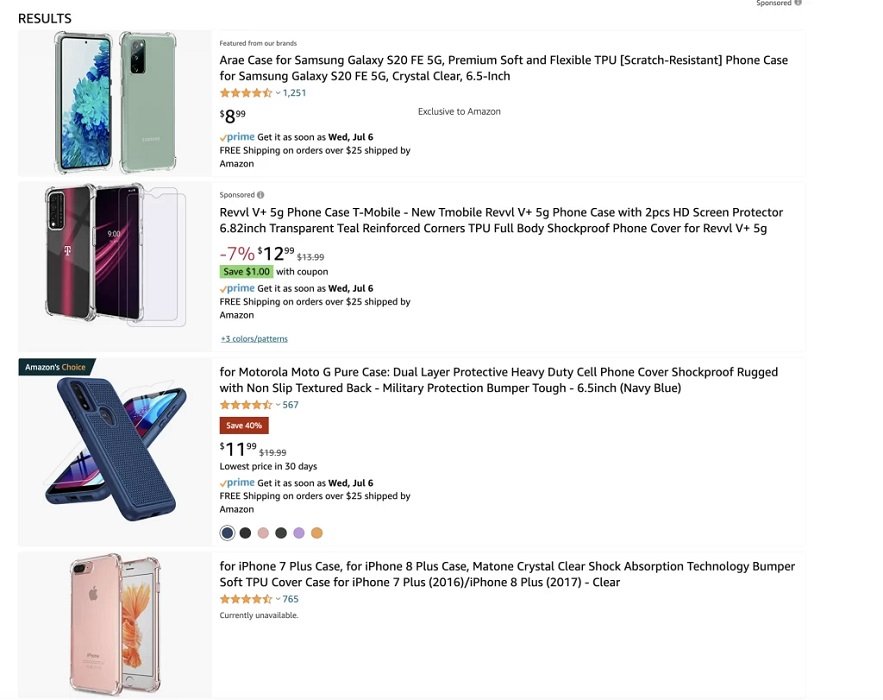This image is a screenshot from the website Selvia.com, showcasing popular phone cases available for sale, each aimed at top niches that could potentially drive significant sales on Amazon in 2022. The screen displays detailed information about four distinct phone cases:

1. **Samsung Galaxy S20 FE 5G Red Case**:
   - **Type**: Premium Soft and Flexible TPU Scratch-Resistant Case
   - **Compatibility**: Samsung Galaxy S20 FE 5G, 6.5 inch
   - **Reviews**: 1,251 reviews, averaging 4.5 stars
   - **Price**: $8.99 on Amazon Prime, available for free shipping on orders over $25, with delivery as soon as Wednesday, July 6th.
   - **Additional Info**: Scratch-resistant and exclusive to Amazon.

2. **T-Mobile Revvl V+ 5G Phone Case**:
   - **Type**: Transparent Teal Reinforced Corners TPU Body Shockproof Case with Two HD Screen Protectors
   - **Compatibility**: T-Mobile Revvl V+ 5G, 6.82 inch
   - **Price**: $12.99 (7% off from original price), save $1 with coupon
   - **Prime**: Free shipping on orders over $25, with delivery as soon as Wednesday, July 6th.
   - **Additional Info**: Available in three different colors and patterns.

3. **Motorola Moto G Pure Case - Amazon's Choice**:
   - **Type**: Dual Layer Protective Heavy Duty Cell Phone Cover with Shockproof Rugged Design and Non-Slip Textured Back
   - **Compatibility**: Motorola Moto G Pure, 6.5 inch
   - **Reviews**: 567 reviews, averaging 4.5 stars
   - **Price**: $11.99 (40% off from the original price of $19.99, lowest price in 30 days)
   - **Prime**: Free shipping on orders over $25, with delivery as soon as Wednesday, July 6th.
   - **Additional Info**: Available in six different colors.

4. **iPhone 7/8 Plus Case - Matone Crystal Clear Bumper**:
   - **Type**: Soft TPU Cover with Shock Absorption Technology
   - **Compatibility**: iPhone 7 Plus 2016 / iPhone 8 Plus 2017
   - **Reviews**: 765 reviews, averaging 4.5 stars
   - **Price**: Currently unavailable
   - **Additional Info**: Features a crystal clear design with bumper protection.

The right-hand side of the screen features images of these phone cases on their respective phones, while the left-hand side provides comprehensive descriptions and specifications for each product.